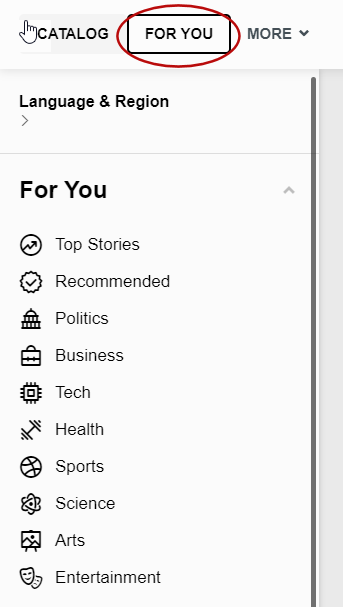The image features a gray background at the top, with the text "CATALOG FOR YOU AND MORE" displayed in black capital letters. On the right side of this text, there is a drop-down menu button. The section labeled "FOR YOU" is highlighted with a black box, which is further accentuated by a red oval encircling it.

Below this, the text "Language and Region" is displayed, followed by a greater than symbol. A thin gray horizontal line extends across the width of the section, with a vertical black line on the far right side, resembling a scroll bar.

Underneath the horizontal gray line, the following categories are listed in order:
- For You
- Top Stories
- Recommended
- Politics
- Business
- Tech
- Health
- Sports
- Science
- Art
- Entertainment

Each category is clearly separated, providing a structured and organized view of the different sections available.